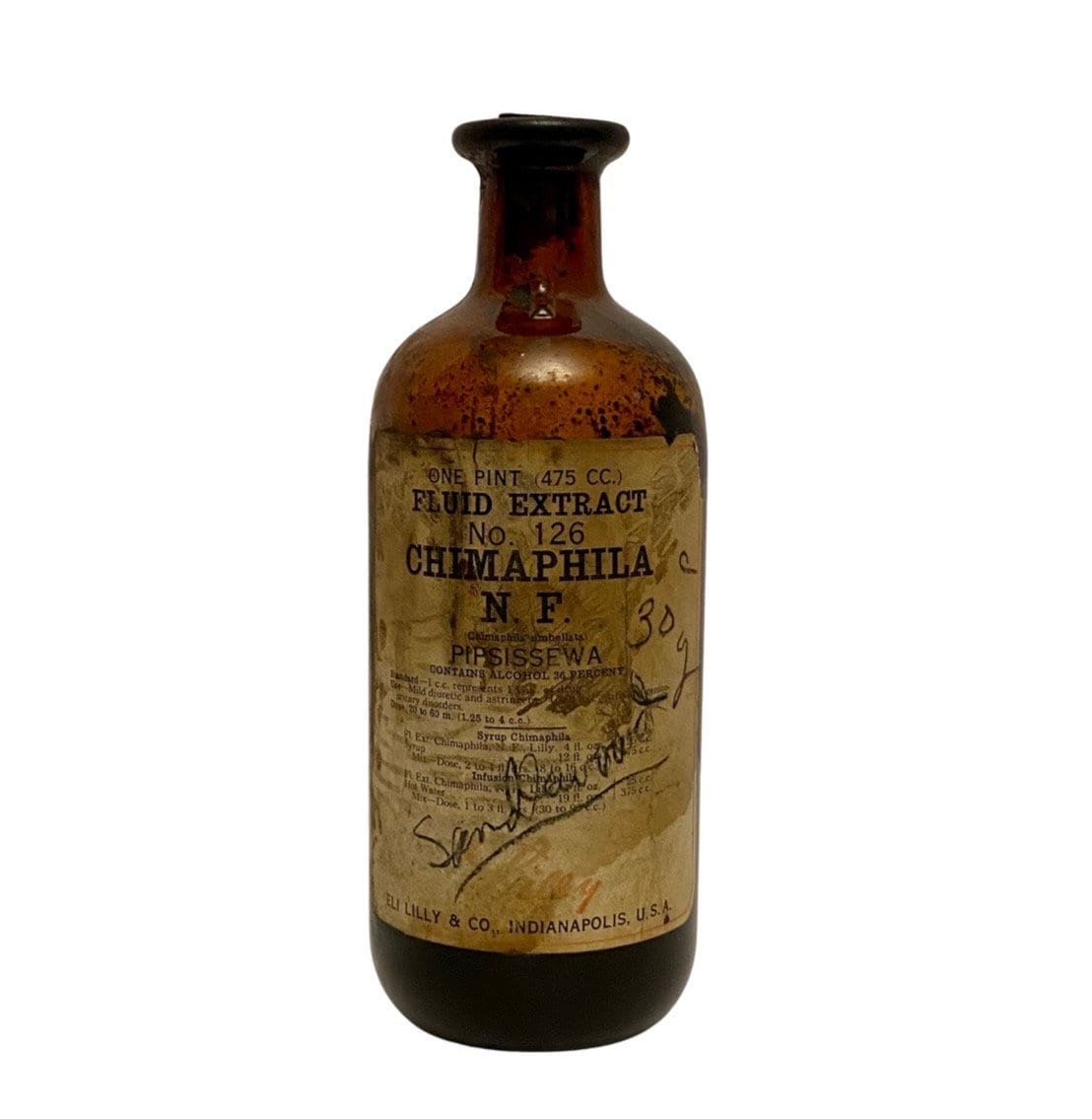The image showcases an antique amber-colored glass bottle set against a plain white background. The bottle, which appears well-worn and is speckled with black splotches, features a neck approximately an inch tall that flutes out to the top. The bottle is adorned with an old, torn beige label now stained brownish from age. The label displays the text "One Pint 475 CC Fluid Extract Number 126 CHIMAPHILA N.F." in black lettering. Below this, the label indicates "Contains Alcohol 36% Syrup" and the producer, "Eli Lilly and Co. Indianapolis, USA." Handwritten in black cursive on the label is the word "Sandalwood," which is underlined and written diagonally near the bottom. Other handwritten notes include "30 grams" scribbled on the side.